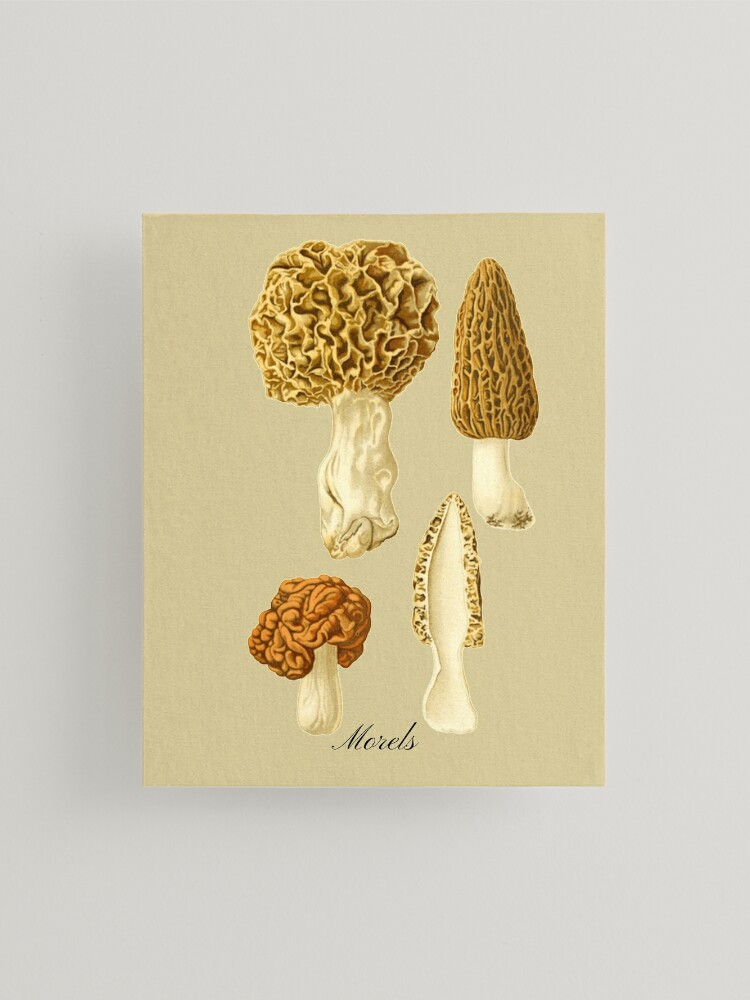This photograph captures a detailed painting of morel mushrooms displayed against a slightly off-white wall. The painting, centered in the image, showcases intricate and somewhat realistic depictions of four morel mushrooms arranged in a quadrant on a beige, presumably canvas background. 

The upper left mushroom is larger with a rounded, bulbous cap exhibiting a dark orange to light orange swirly pattern atop a whitish, cream-colored stem. To its right, the upper right mushroom features a conical shape with similar coloration and a cream-colored stem with darker shading. On the lower left, there is a smaller specimen with a dark orange and orange irregular, brain-like cap, and a whitish stem with cream shading. Finally, the lower right quadrant shows a vertical cross-section of a conical-shaped morel, revealing a cream-colored interior and stem accented by orange and dark orange on the exterior. 

Below the artwork, in script font, the word "MORELS" is inscribed, identifying the mushrooms. The artistic style is precise yet painterly, resembling illustrations found in encyclopedias or botanical texts.